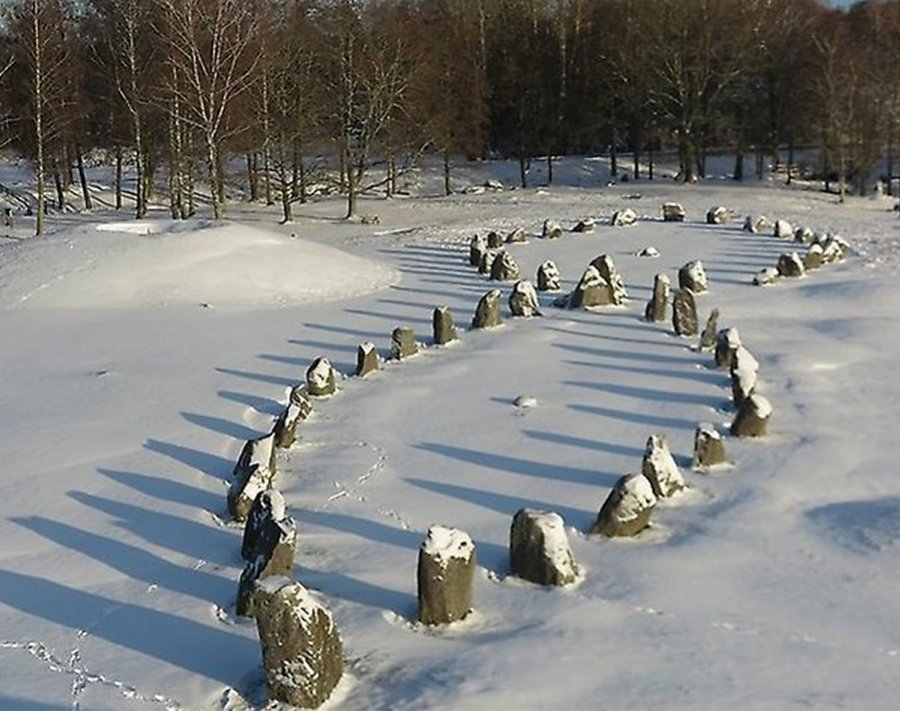The photograph captures a serene, wintry outdoor scene dominated by a blanket of snow. At the heart of the image lies a meticulously arranged rock formation, shaped into a clear figure-eight pattern, with each rock protruding above the snow and topped with a light dusting. This central pattern appears too deliberate to be natural, suggesting human placement. Surrounding the formation, the ground is thoroughly covered in snow, featuring various animal tracks, likely from small creatures such as rabbits and squirrels.

On the left side of the image, there is a prominent mound of snow with a noticeable hole at its top. Footprints can be seen dispersed across the snowy terrain, leading towards the figure-eight structure. In the distance, a road runs along the top of a bank, possibly crossing a small creek suggested by a faint indentation in the snow.

The background is lined with a mix of leafless deciduous trees typical of winter, with a few darker, evergreen trees interspersed. The absence of leaves and the low position of the sun, casting elongated shadows, indicates that it is late in the day. The peaceful, snowy landscape is devoid of any visible text or human-made markers, emphasizing the natural beauty and contemplative solitude of this winter scene.